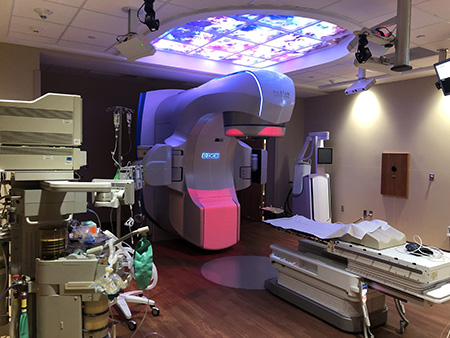This photograph depicts a detailed view of a medical facility room designed for imaging procedures. Dominating the center of the room is a large, multi-colored medical imaging machine. The main body of the device is primarily gray and white, adorned with subtle pink accents at the bottom, and features a distinctive gray hood with a projection extending from it. Directly in front of the imaging machine is a padded gurney or medical table, equipped with a paper sheet and a section for leg placement, indicating where a patient would lie down for imaging scans.

The room's aesthetic includes white walls and wooden flooring, and it is illuminated by a drop ceiling with a striking stained glass window directly above the imaging machine. This stained glass window, adorned with blue and pink hues, casts colorful reflections onto the equipment below. To the left side of the room, additional medical apparatus is visible, although its specific functions are not entirely clear from the image. This section also includes a chair and a desk, likely part of a viewing station for medical personnel to evaluate the images produced by the machine. The overall setting is indicative of a sophisticated, well-equipped medical environment.